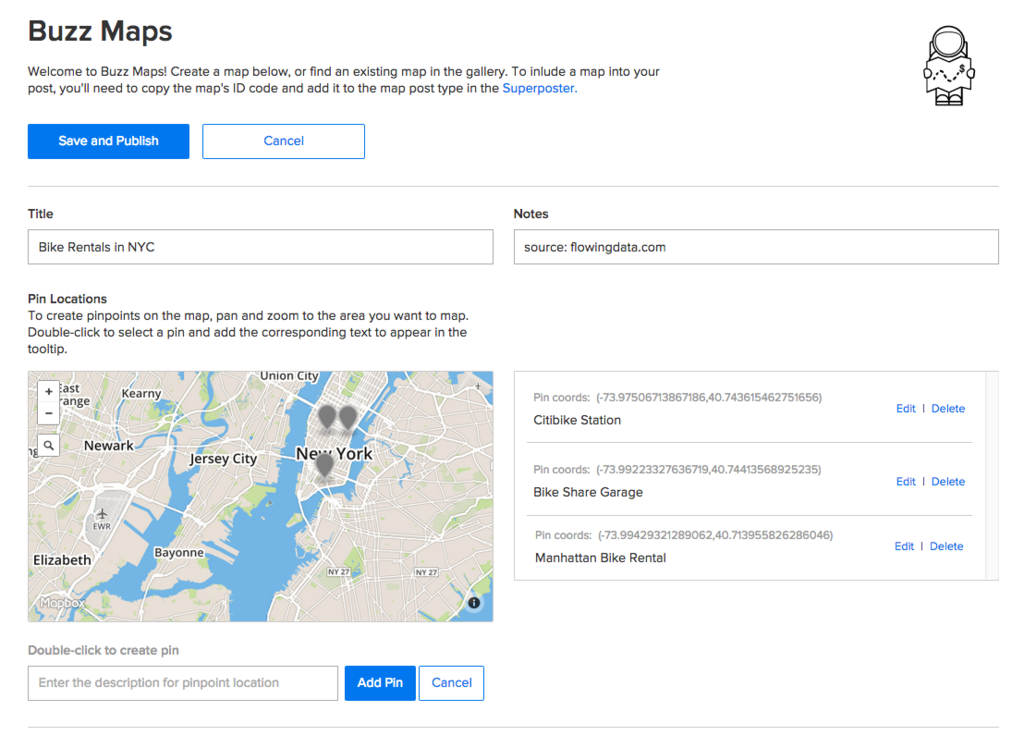In the upper left corner of the image, the title "Buzzmaps" is prominently displayed. Below it, a welcoming message reads, "Welcome to Buzzmaps. Create a map below or find an existing map in the gallery." The instructions continue, advising users to copy a map's ID code and add it to the map post type in a "super post" section, which is highlighted in blue.

On the right side, an illustration of an astronaut holding a map icon is visible. Beneath this graphic are two buttons: "Save and Publish" in blue with white text, and "Cancel," which is white with blue text and outlined in blue. A dividing line separates these elements from the next section.

Below the line is a title input field displaying "Bike Rentals in New York City." Additional input fields include "Notes" with the source noted as "flowingdata.com," and "Pin Locations." Users are instructed to pan and zoom the map area to locate their desired points. Double-clicking a location allows the user to place a pin and add corresponding tooltip text. Current pins are placed on New York City, New Jersey, and Newark, with three gray pins marked on New York Island.

At the bottom of the interface, there is a prompt to double click to create a new pin, accompanied by a data box for entering a description for the pin location. Options to "Add Pin" and "Cancel" are available, providing a clear, streamlined process for map creation and editing.